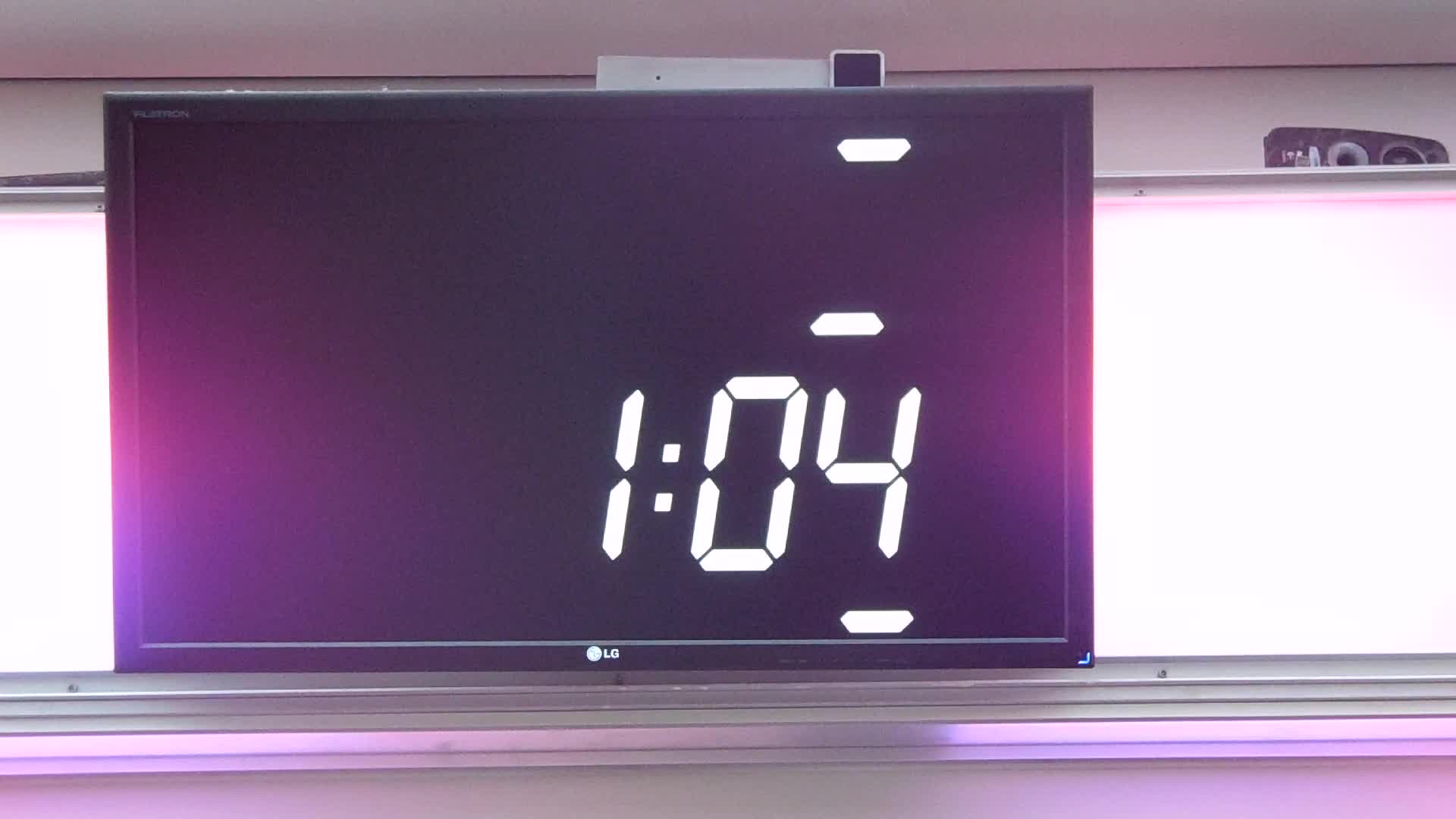This detailed photograph captures a close-up of what appears to be an electronic device, likely a tablet, featuring a sleek and modern design. The rectangular device is dominated by a dark purple screen that prominently displays the time "1:04" in large, bold numbers. The screen is bordered by several horizontal bars; the topmost is a light lilac, followed by a white section on each side, and then another gray bar. Another lilac bar is situated below the gray one. Above and below the time are thin white lines, with an additional white line located in the upper right corner. At the bottom center of the device, the brand logo "LG" is clearly visible, hinting at its origin. A light lilac bar tops the display, contributing to a visually appealing and structured layout in the overall design.